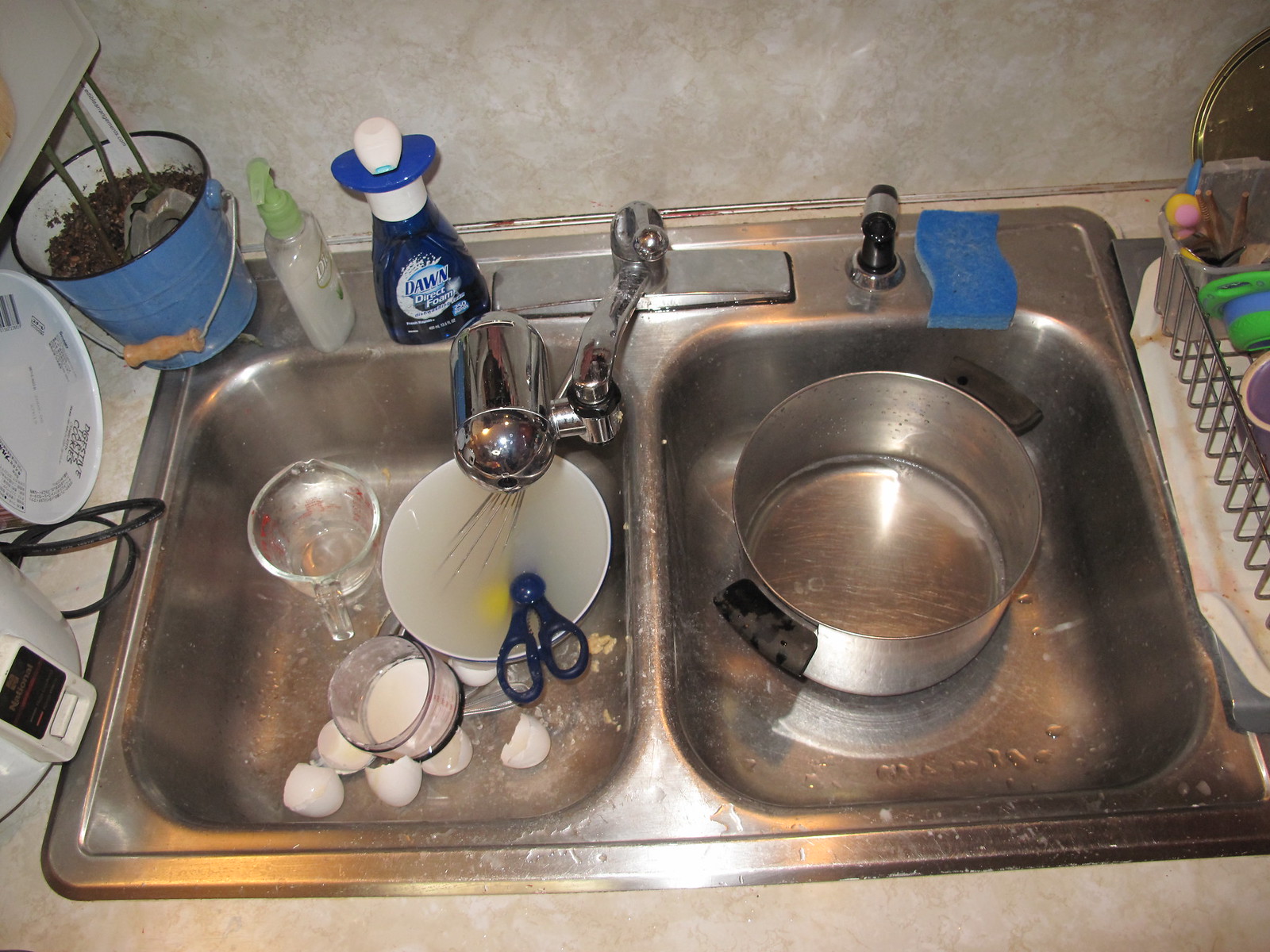This horizontal color photograph showcases a typical kitchen scene centered around a double stainless steel sink with a matching metal faucet. The right side of the sink houses a large pot awaiting a thorough wash. On the left side, a collection of items needs cleaning: a bowl containing a pair of scissors, a glass or plastic measuring cup, another bowl with remnants of white liquid, possibly milk, and cracked eggshells scattered within the sink. 

Adjacent to the sink on the countertop, a blue sponge featuring both a scrubbing and a soft side lies ready for use. A convenient pull-out sprayer is attached to the sink for easy rinsing. Nearby, a bottle of Dawn dish soap stands alongside what appears to be Dial hand soap. Additionally, there's a small pot, potentially for discarding vegetable scraps. To the right of the sink, a drying rack holds freshly washed dishes, positioned so that any excess water can drain directly into the sink.